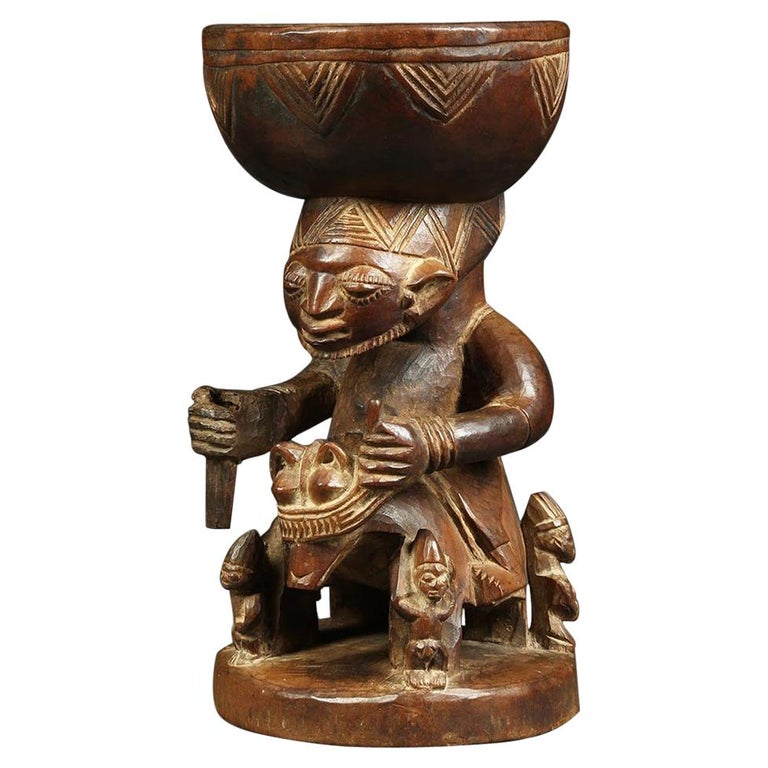This image depicts a detailed, wooden carved statue of a bearded man. The statue, crafted from a dark, shiny wood, has the man seated atop an animal that resembles a dog or a wolf. The man is adorned with a bowl-like hat with triangular accents carved into it, which appears to be balanced on his head. He is holding an indistinct object in his right hand. Surrounding the base of the statue, which is circular, are smaller figures, possibly symbolic guardians or attendants. The intricate detail and design elements suggest that this may be an African tribal artifact.